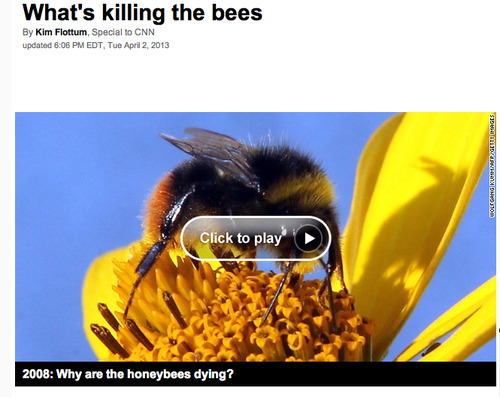This detailed image, associated with the article "What's Killing the Bees" by Kim Flodum, exclusive to CNN and updated at 6:06 PM EDT on Tuesday, April 2nd, 2013, features a visually striking honey bee positioned on a vibrant yellow flower. The accompanying page includes a video link titled "2008: Why Are the Honey Bees Dying?". The honey bee is visibly yellow and black, with a hint of orange towards the rear of its body. Its distinct wings are perched atop its body, and the bee's stinger and legs are clearly depicted. The flower itself boasts a bright yellow center surrounded by matching yellow petals. Notably, the bee casts a shadow onto one of the petals, adding depth and dimension to the image.